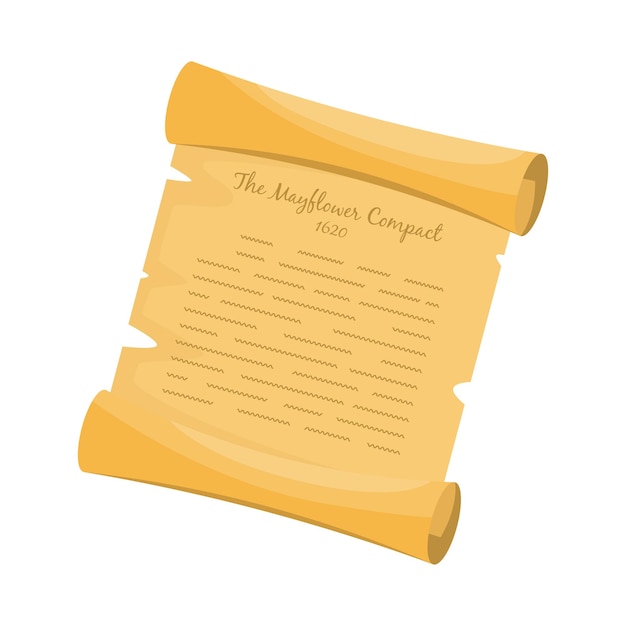This detailed image is a graphical computer-drawn illustration of a historically-themed scroll, set against a clean white background. The scroll, depicted in light beige with slight yellowed patches along the damaged, torn edges, is unfurled to display its contents. It is positioned at a slight diagonal angle, with the right side closer to the viewer. Both ends of the scroll remain partially curled, revealing a bit of paper within the single curl. The scroll exhibits signs of wear, with intermittent curved triangular cuts along the sides, enhancing its weathered appearance. The top of the scroll bears the italicized title "The Mayflower Compact," followed by the date "1620" in the middle section. Below these titles, in place of actual text, are squiggly lines arranged like a heartbeat monitor, running horizontally down in a single paragraph to suggest the presence of written content. This stylized representation, with its detailed nuances in shading and texture, evokes the appearance of an aged, significant historical document.